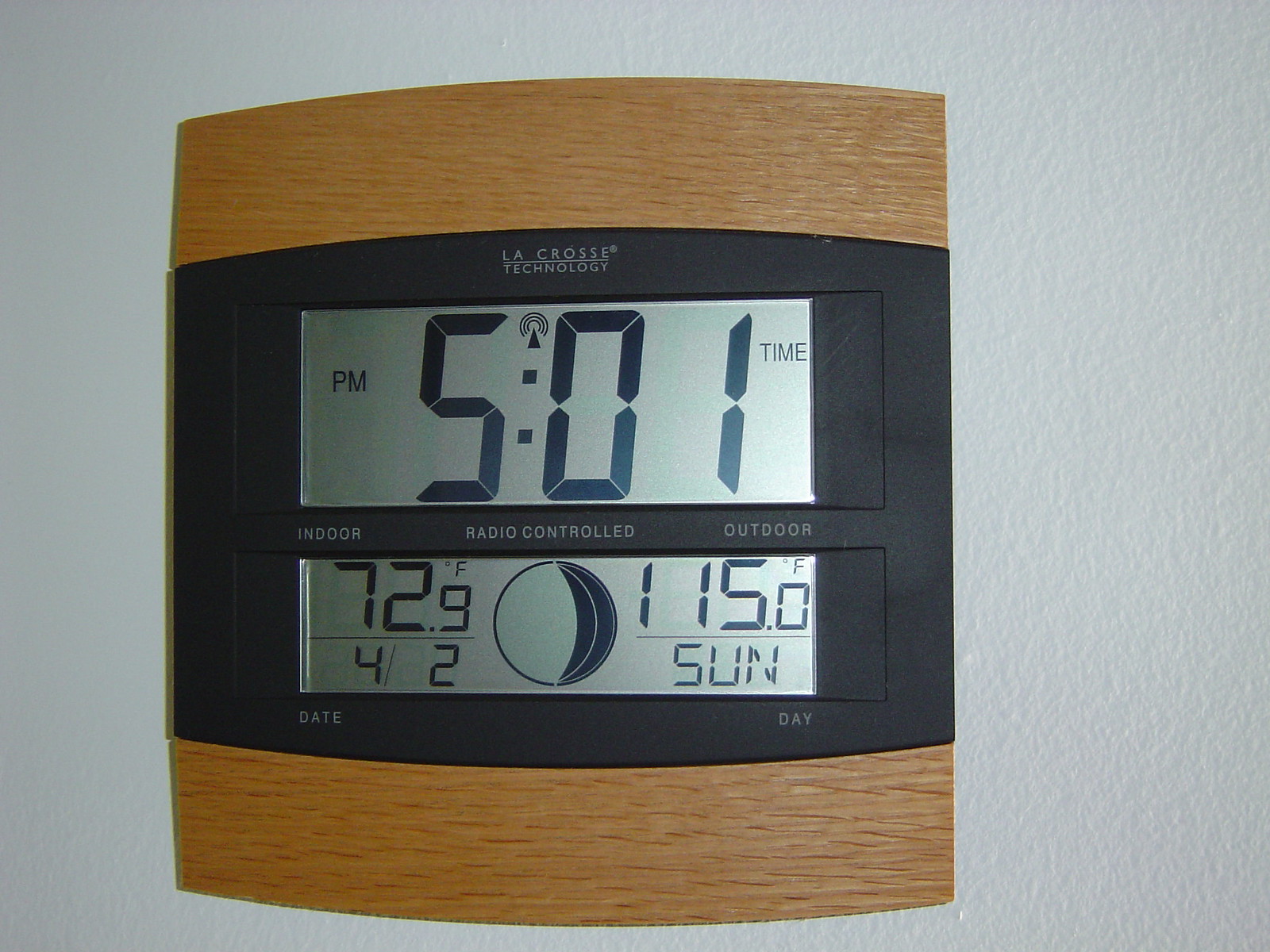The image showcases an off-white, textured wall that gives a bumpy appearance akin to goosebumps on an arm. The wall appears darker on the left side due to shading, while the right side is lighter. Dominating approximately 75% of the image is a clock with a unique design. The clock has a wood grain finish on both the top and bottom edges, while the middle portion is made of black plastic. Its shape is almost square, but the top and bottom edges are slightly rounded.

At the top of the black section, in white lettering, it reads "La Crosse Technology" with a line separating "La Crosse" and "Technology." Below this text is a silverish-green LED screen displaying the time, which reads "5:01 p.m." in large numerals. In small letters, the word "time" is noted towards the upper right of the time display.

Further down, the black section contains the words "Indoor," "Radio Control," and "Outdoor" from left to right. Below this text, another silverish-green screen presents the indoor and outdoor temperatures: 72.9°F and 115.0°F, respectively. Additional details include "4-2" on the screen's bottom left corner and "Sun" for Sunday on the bottom right. In the center, there is an icon resembling a circle or moon, indicating the current moon phase.